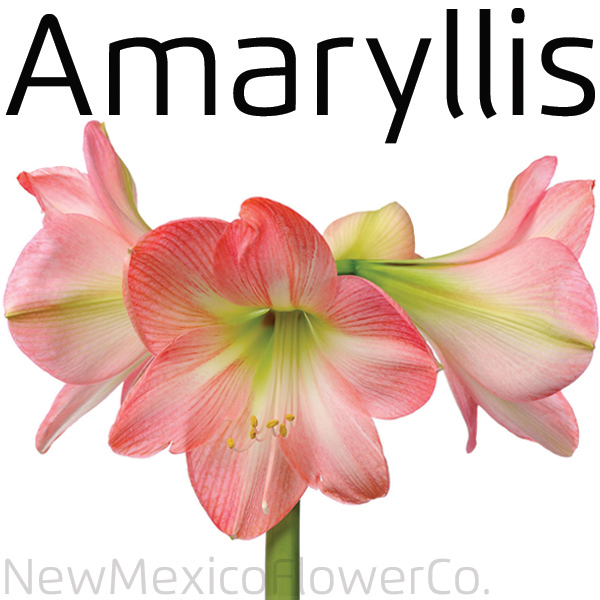The image features a striking pink amaryllis flower prominently set against a solid white background. Centered at the top in large black letters, the text "Amaryllis" (A-M-A-R-Y-L-L-I-S) stands out. The flower, which appears to have four visible petals, displays a mix of dark pink and light pink stripes, with the petals becoming richer in color towards the edges and tapering off to a lighter tint near the center. The middle of the flower boasts a greenish-yellow hue, with tiny seeds emerging from it. One petal faces directly outward, while additional petals open towards the left and right. There is also a hint of a fourth petal behind the central blossom, adding depth to the image. Emerging from the base of the bloom is a single green stem. Positioned at the bottom of the picture, the text "New Mexico Flower Co." is written in a continuous, unspaced format.